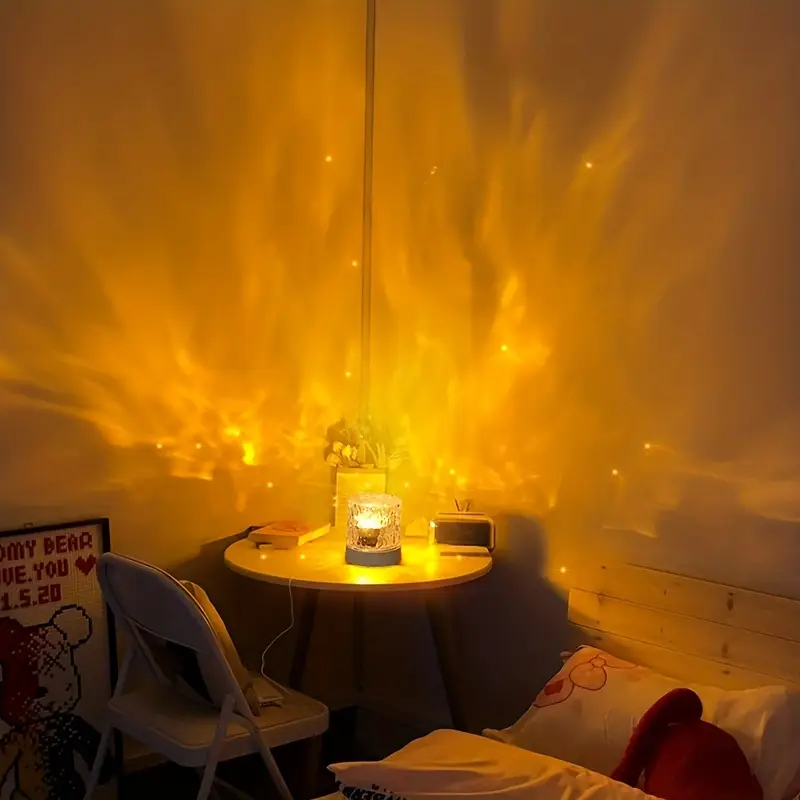This photograph captures a cozy bedroom corner with a variety of distinct and detailed elements. Central to the image is a white table with three black legs, upon which sits a notable light fixture with a rounded gray base and a crystallized cylindrical body. The light in the center of this fixture emits a warm yellow to white glow, casting intricate patterns on the walls reminiscent of flickering firelight. This dynamic illumination creates a captivating atmosphere in the room.

To the left of the table is a gray metal folding chair. Leaning against the wall beside this chair is a framed, crocheted poster featuring a stylized teddy bear with black X's for eyes. The top of the poster includes partially visible text that reads "My Bear, you [heart symbol] 1.5.20," hinting at a sentimental message.

On the table, alongside the light fixture, is a small ensemble of items including what appears to be an alarm clock, a book, and a bag. A cable extends from the table, likely connecting to the light fixture that creates the mesmerizing light patterns. In the bottom right corner of the image, part of a bed with a wooden headboard can be seen, adorned with a white pillow featuring a pink bow design.

This charming and detailed bedroom scene evokes a sense of warmth and personal history through its thoughtfully arranged objects and ambient lighting.